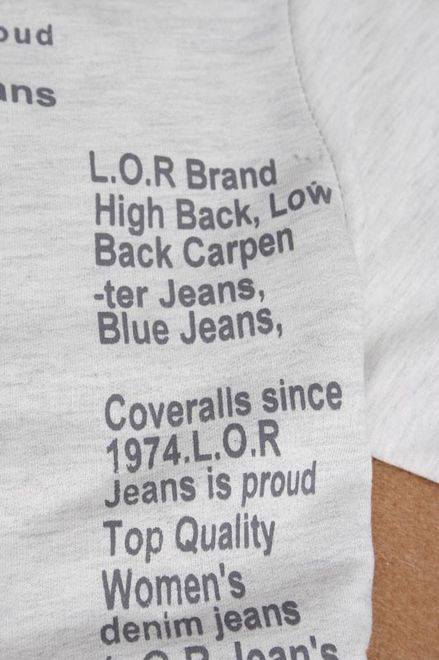This detailed photograph captures a close-up view of a gray fabric which appears to be part of a shirt or similar garment, possibly made of t-shirt or sweatshirt material. The fabric is positioned against a medium brown, porous surface, likely corkboard or carpet. The visible portion of the garment, identified as the front left side near the armpit or sleeve seam, features black text running vertically along the fabric. The text includes several lines, reading: "LOR brand high back low back carpenter jeans blue jeans coveralls since 1974 LOR jeans is proud top-quality women's denim jeans." While some additional words exist in the upper left corner, they are not fully visible in the frame. The right edge of the fabric cuts off part of the text, leaving the remaining lines out of view.